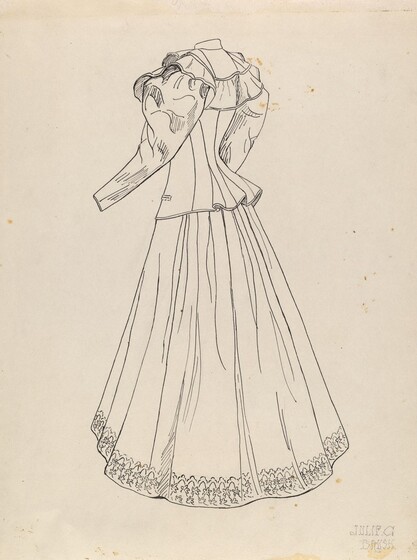This is a rectangular image taller than it is wide, featuring a meticulously detailed pencil or ink drawing on aged, cream-colored manila paper, which is marred by several brown, rust-like and dirt-like spots. In the bottom right corner, there is a faint, small signature that appears to read "Julie G. Burris." The drawing is a black-and-white depiction of a fancy, early 1900s dress viewed from the back, showcased on a headless mannequin. The dress, characterized by its long, flowing skirt that reaches the ground, features intricate embroidery along the hem and a petticoat underneath. The garment includes long sleeves with slim wrists, elaborate ruffles or gathers around the neck, and additional ruffles cascading down the back. The back of the jacket is detailed with multiple seams and a square cutout, while the sleeve tops are puffy, tapering down to the wrists. This highly detailed image captures not only the beauty of the dress but also the texture and aging of the paper on which it is drawn.